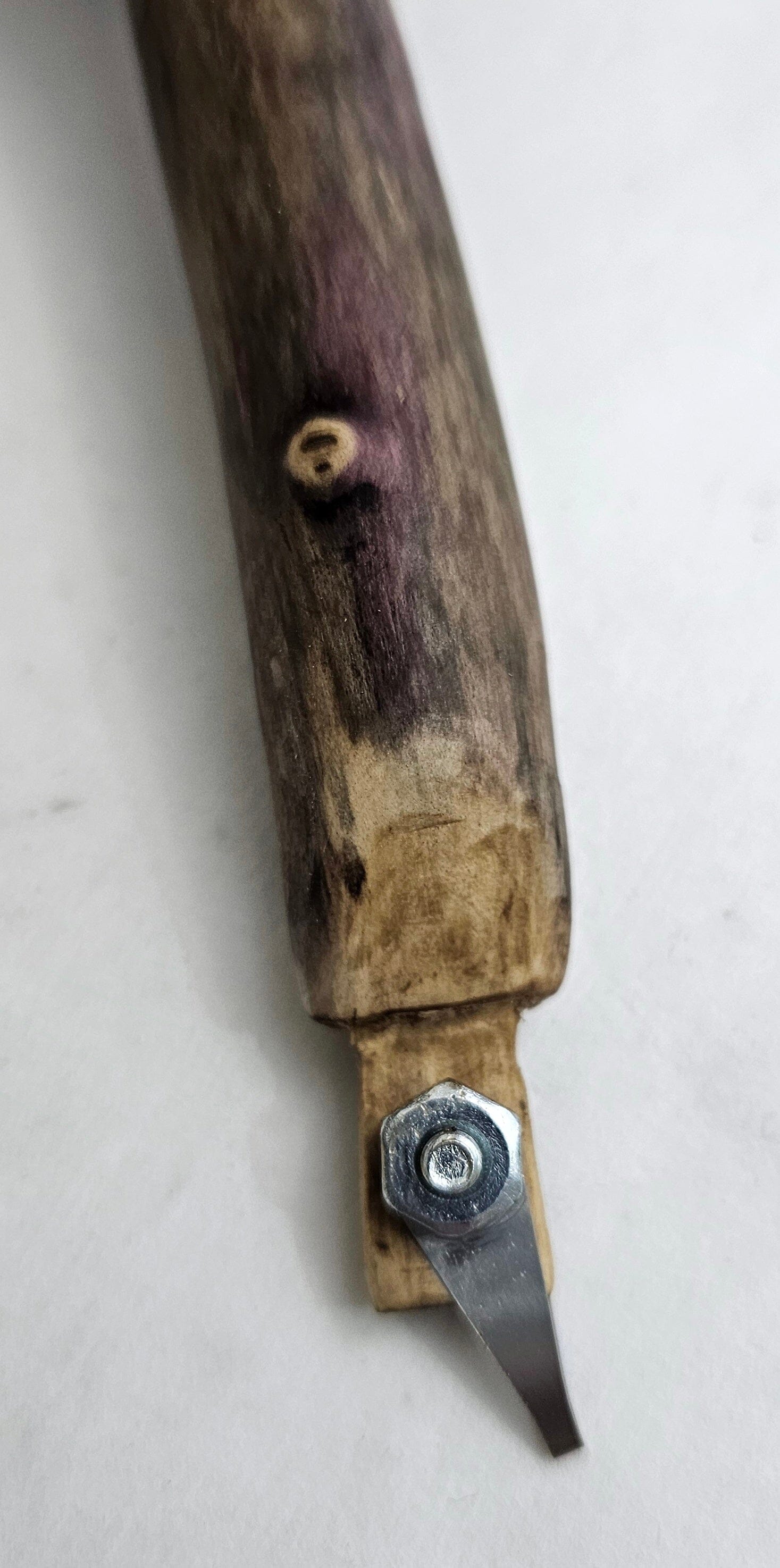The image is a color photograph on an off-white background depicting a homemade tool crafted from a tree limb. The wooden shaft, brown from staining, shows clear whittle marks and grain patterns, including a spot that might be a knot. Its handle extends beyond the frame, suggesting it is fairly long. The end has been meticulously whittled down to form a flat and rounded area where a small, chisel-like metal piece is attached. This metal piece is secured by a bolt and nut, protruding from the flat end of the wood, and features a squared-off tip. The tool, possibly used for tasks such as trimming or cutting, is clearly handmade and exhibits detailed craftsmanship.